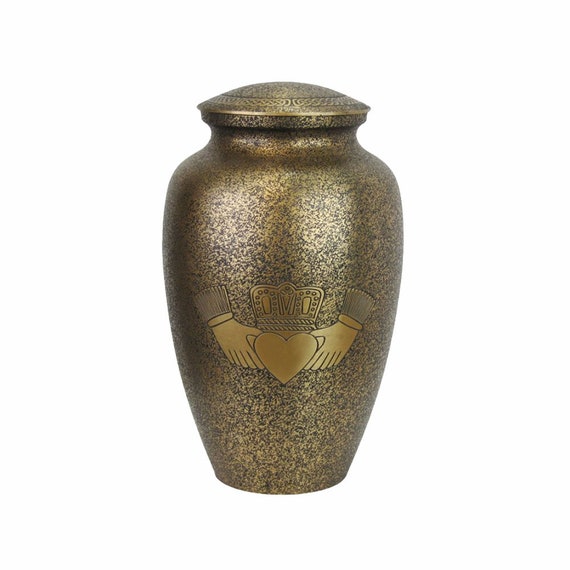The image showcases a large 3D urn set against a solid white background, creating no clear separation between the background of the page and the picture. The urn itself is brass-colored with a speckled design, intertwined with shades of black and dark gray. Prominently featured on the front is a Claddagh symbol: two hands emerging from gray sleeves hold a golden heart, topped with a golden crown. Delicate black lines and decorations accentuate the heart and crown, making the Claddagh image stand out vividly against the urn's surface. Additionally, a Celtic scroll-like pattern encircles the top rim, adding an elegant touch. The urn, made of brass and sizeable enough for the crematory remains of a pet, is both lovingly decorated and visually striking.